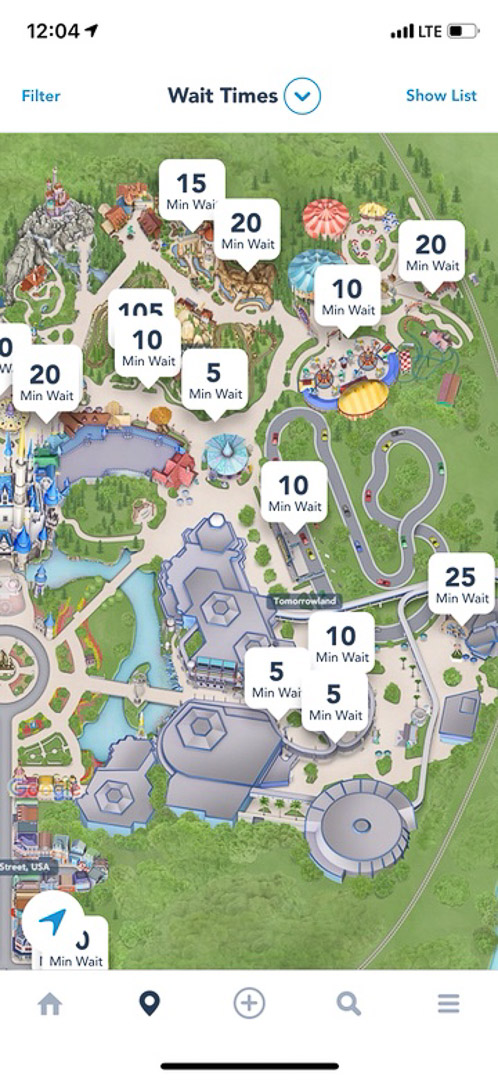This image is a detailed screenshot of a city-building game interface. 

At the top of the screen, it displays "12:04" in black text along with a small black icon resembling a paper plane on one side. On the opposite side, there is an "LTE" label indicating the network type, alongside a signal strength indicator and a battery icon that appears about half full, with no percentage displayed. 

The upper part of the interface features options in blue text: "Filter" and "Wait Times," flanked by a clickable blue circle with a downward arrow. Another blue-linked option reads "Show List."

Centered in the image, there is an aerial view of the virtual city map. The landscape showcases numerous white boxes with black text inside them, each signifying various wait times for different attractions or activities, ranging from five minutes to potentially a hundred and five minutes. 

Spanning the city, you can see greenery with light green grass and bodies of water. The area includes grey circular structures interconnected by roads, a prominent grey castle with a flag, and a colorful carnival area characterized by a red and white circus pattern. Scattered throughout the cityscape are several colored cars in shades of yellow, blue, and red, along with green bushes.

Towards the bottom of the screen, there's a blue paper airplane icon within a white circle and additional interface icons. These include a grey house, a black location pin, a grey circle with a plus sign, a grey magnifying glass, and some grey lines. Below these icons is a thin black line, marking the lower boundary of the interface.